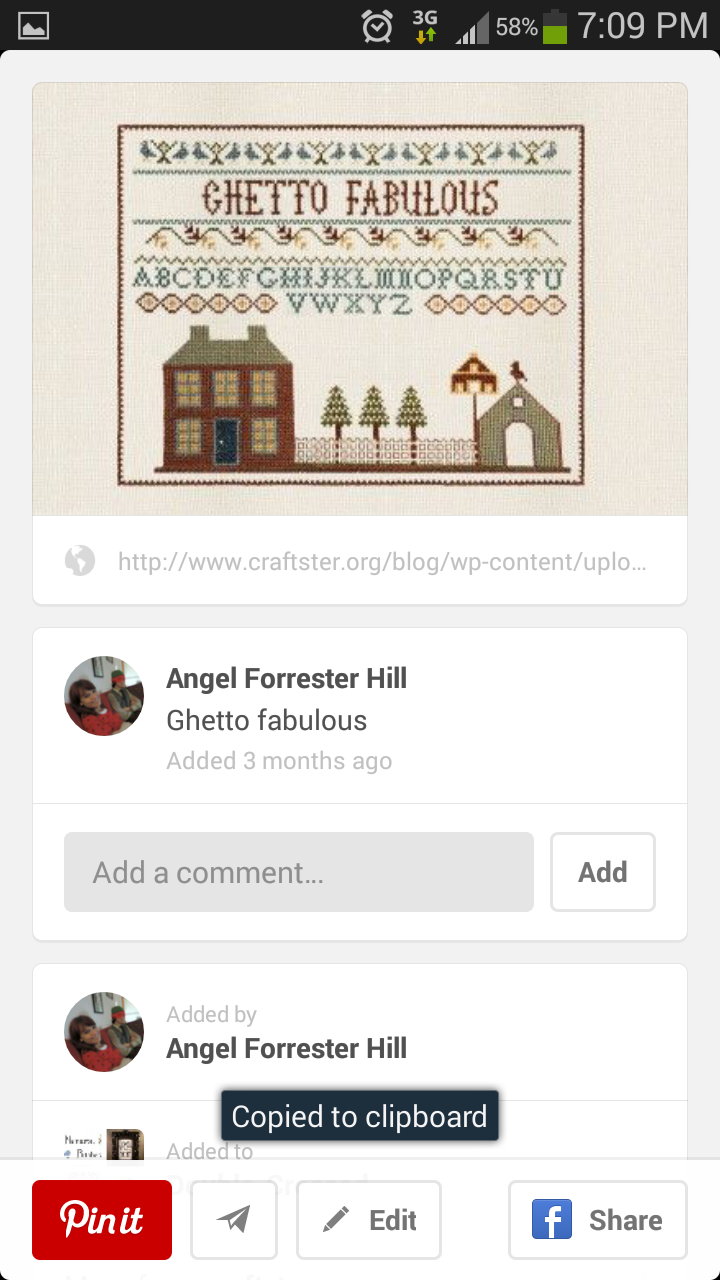The image, a screenshot from a mobile device, showcases an intricate needlepoint artwork uploaded by Angel Forrester Hill to a social media site, likely Pinterest. The top portion of the image features colorful quilt-like embroidery that reads "Ghetto Fabulous," including the alphabet A through Z. Also depicted are houses with fences, a barn with a weathervane, and several trees in varying shades of red, green, blue, tan, white, black, and gray. Below this artwork, the user "Angel Forrester Hill" is named, along with the duplicate text "Ghetto Fabulous." The bottom left includes a "Pin it" button, while the bottom right holds a "Facebook Share" button. The mobile interface shows additional icons like a photo icon, an alarm, a 3G signal bar, battery percentage, and a timestamp. The URL leading to the needlepoint image is "http://www.craftster.org/blog/wp-content/uploads". Users are given options to copy the image link to clipboard, pin it, edit, and share on Facebook.